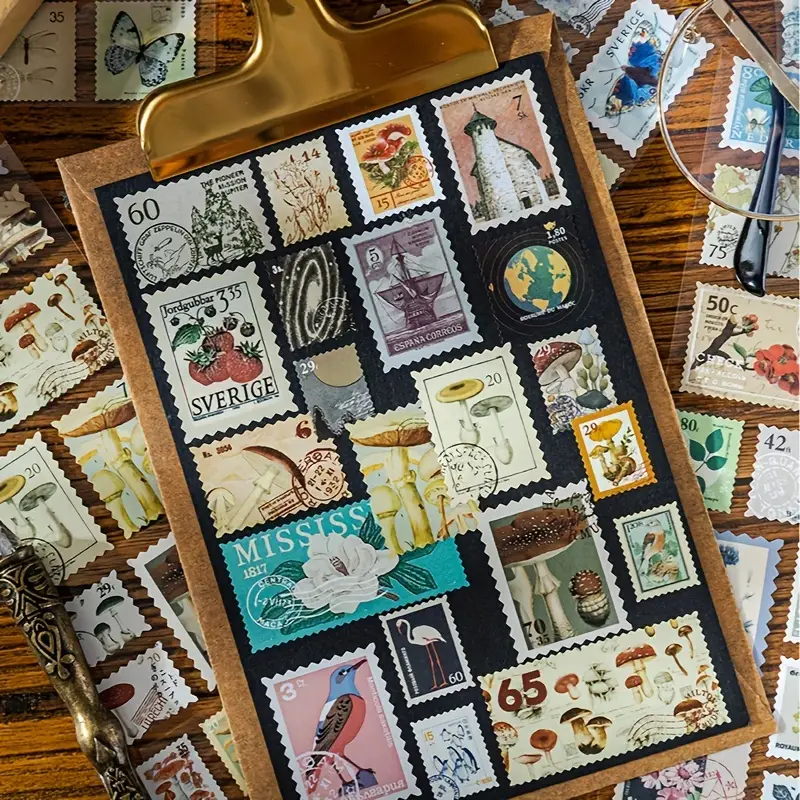The image depicts a rectangular clipboard with a gold clip at the top, positioned slightly taller than it is wide. The clipboard, which has a brownish, golden appearance resembling a corkboard, holds a black sheet displaying an eclectic assortment of stamps. Among these stamps, notable designs include mushrooms, a barn, a black and white bird, strawberries with the word 'Severage', and a stamp from Mississippi dated 1817 with a flower. Surrounding the clipboard, there are additional clear pages or folders also showcasing stamps. All these items are laid out on a wooden table with a medium green wood tone, providing a cohesive backdrop to the stamp collection.